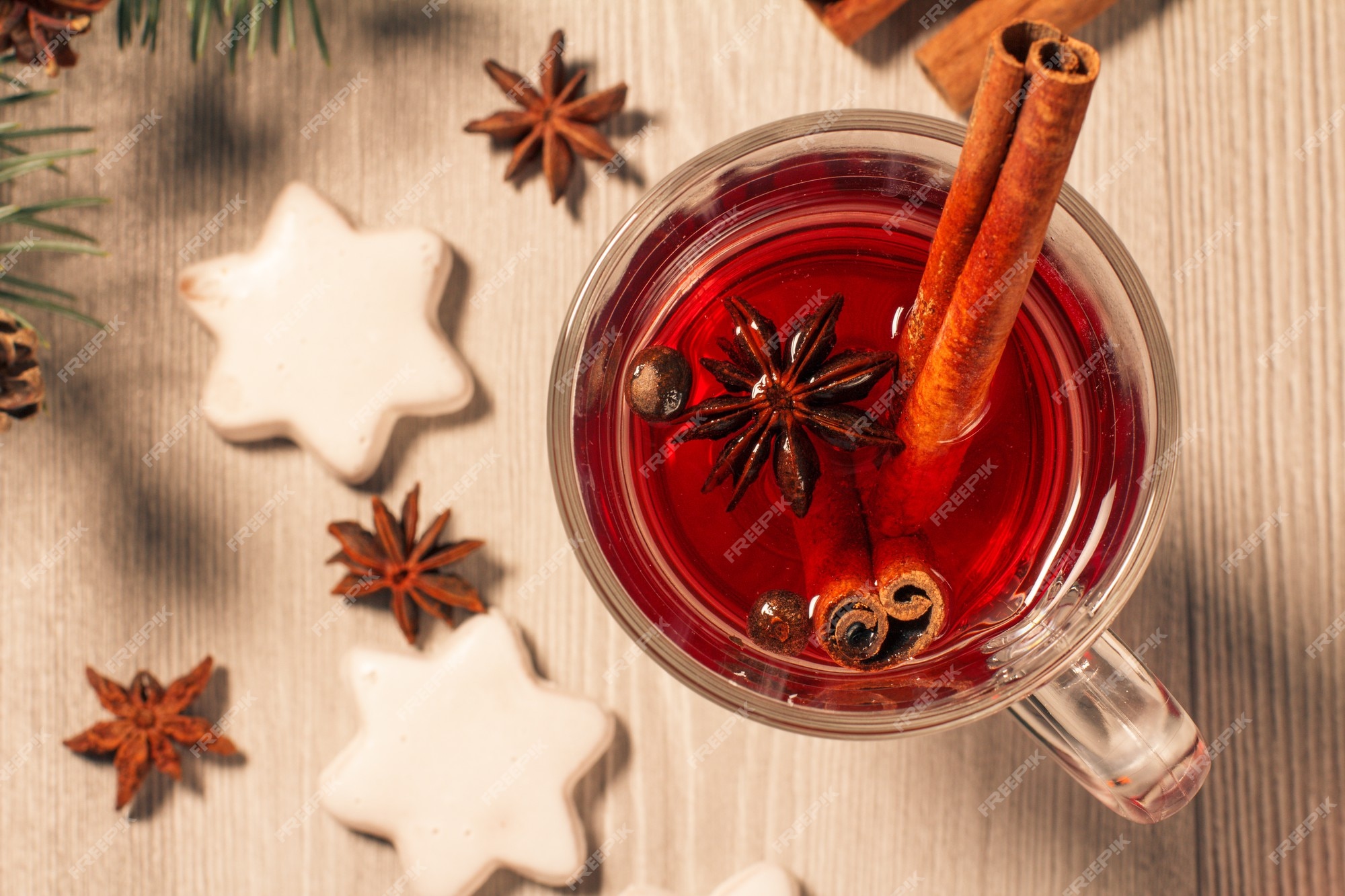The photograph, taken indoors, looks straight down on a clear glass cup filled with a reddish-colored liquid, likely cider or tea, resting on a light brown wooden table with visible grain and vertical slats. The cup is positioned towards the right-hand side, with a handle pointing to the bottom right of the image. Inside the cup, amidst the red liquid, floats a full piece of star anise and a couple of cinnamon sticks, partially submerged.

To the left of the cup, there are three more pieces of star anise scattered on the table, along with two prominently displayed six-pointed star-shaped cookies adorned with white icing. Partially visible is a third cookie at the bottom center of the image. In the upper left corner, you can see pine needles, part of a pine cone, and a hint of green foliage, adding a festive touch to the composition. Additionally, a few more cinnamon sticks are visible in the upper right corner of the photograph. The overall scene is one of cozy warmth with a touch of holiday charm.